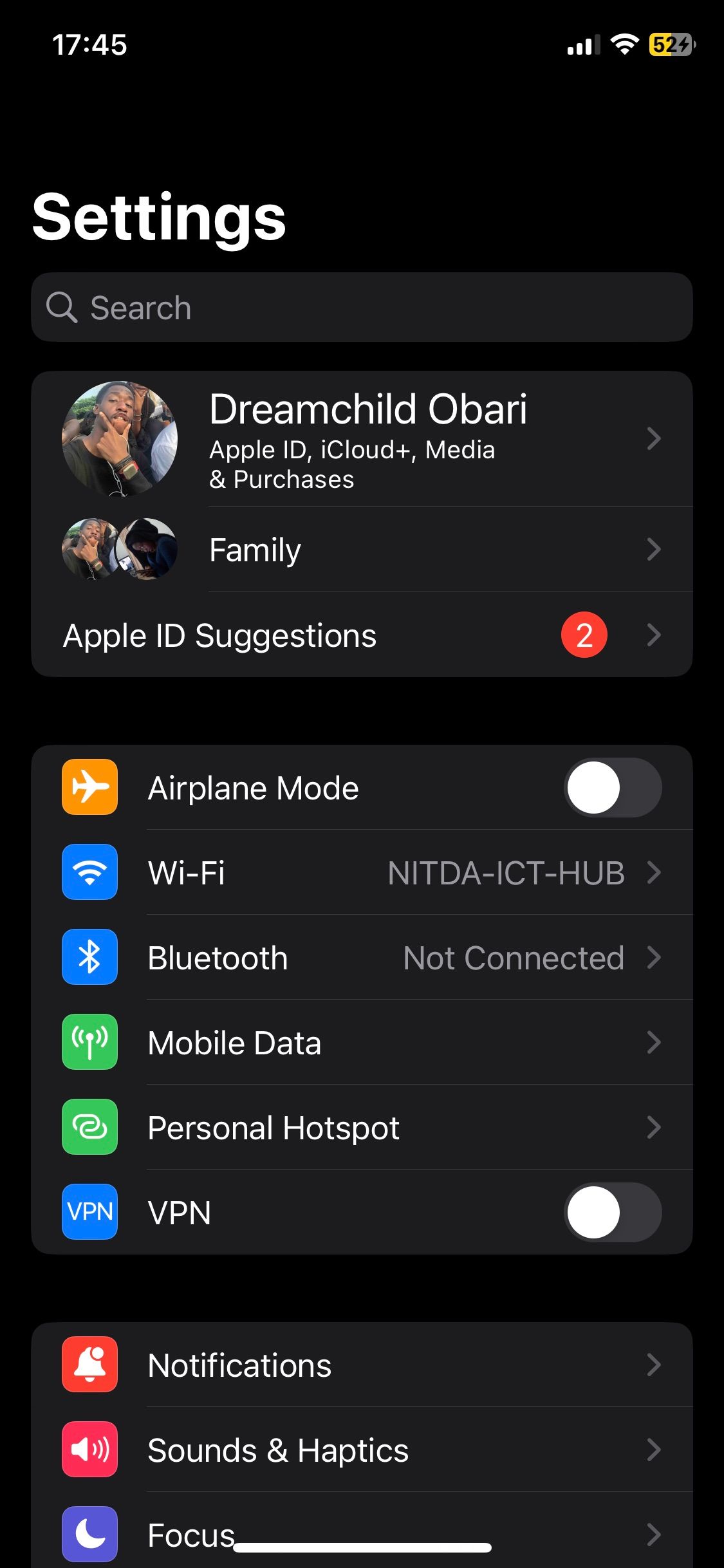The image shows a cell phone screen with a black background. In the top left corner, the time is displayed as 17:45. To the right of the time, there are icons indicating signal bars, Wi-Fi signal strength, and a battery level at 52%. 

Centered below these icons are the words "Settings" in large, bold, white letters. Directly below "Settings" is a search bar. Underneath the search bar, there is a circular avatar image of a young Black male making a thinking gesture, with his index finger and thumb on his chin. To the right of the avatar, it reads "Dream Child Obari."

Beneath the name, in smaller letters, it states "Apple ID, iCloud+, Media & Purchases" with an arrow pointing to the right, indicating more details are available. Below this section is a "Family" section highlighted with a family icon to the left and multiple circular avatars.

Following the family section, there is an "Apple ID Suggestions" section, indicated by a red circle with the number 2 inside it and an arrow pointing to the right.

The next section begins with "Airplane Mode" accompanied by a corresponding toggle button. This is followed by "Wi-Fi", which reads "NITDA-ICT-HUB" to the right. Below Wi-Fi, it shows "Bluetooth" as not connected, followed by "Mobile Data" and "Personal Hotspot." Another option, "VPN," also includes a toggle button for enabling or disabling the feature. 

The subsequent section lists additional settings: "Notifications," "Sounds & Haptics," and "Focus," each with their respective icons.